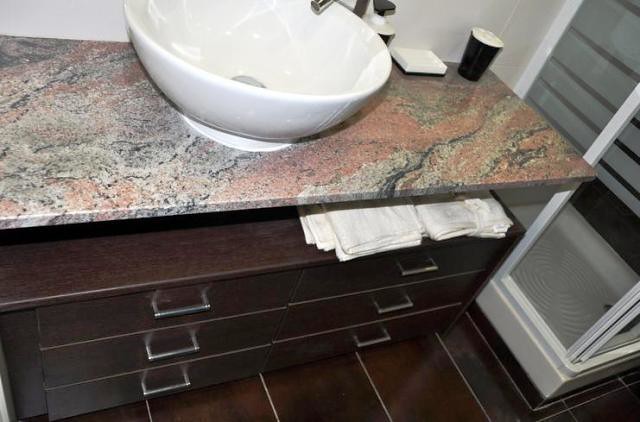A photograph depicts a modern bathroom featuring a unique, bowl-shaped white sink positioned on a sleek drawer unit. The sink, which resembles a large white bowl, is paired with a silver faucet. The drawer unit, topped with polished marble, has six compartments, each with its own handle, providing ample storage space. To the right of the sink, on the marble countertop, sits a black cup and a soap holder. Adjacent to the drawer unit, a predominantly white shower can be seen. The bathroom floor is made of dark brown wood, adding warmth to the space.